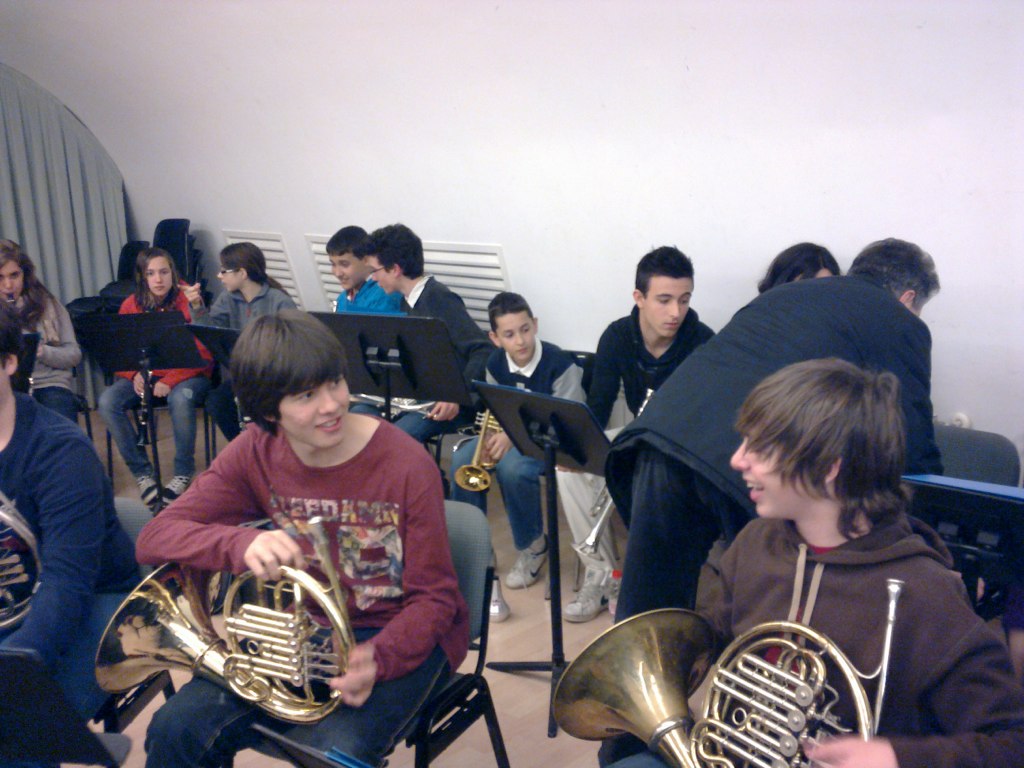In this photograph, a middle school band class is depicted where students around the ages of 10 or 11 are preparing for a music session. The image captures approximately 12 students seated in chairs arranged in front of music stands, indicating a brass and woodwind section. The young boys and girls are engaged in animated conversations, not currently playing their instruments. Two Caucasian boys with dark brown hair are sitting at the front, chatting with each other; one is in a brown hoodie and the other in a navy and maroon long-sleeved shirt, both holding French horns. In the background, more students are holding trumpets and clarinets, while some are simply looking at their music notes. The instructor, dressed in a black jacket and black pants, is seen bending over, likely assisting a student with an unidentified instrument as it is partially obscured by the frame. Among the students, a girl in a grey jacket is pointing something out, conversing with a peer in a red jacket, blue jeans, and black shoes, while another student appears to be blowing her trumpet. This dynamic scene captures the preparatory ambience of a middle school band class, where students are gearing up to play their instruments under the guidance of their teacher.